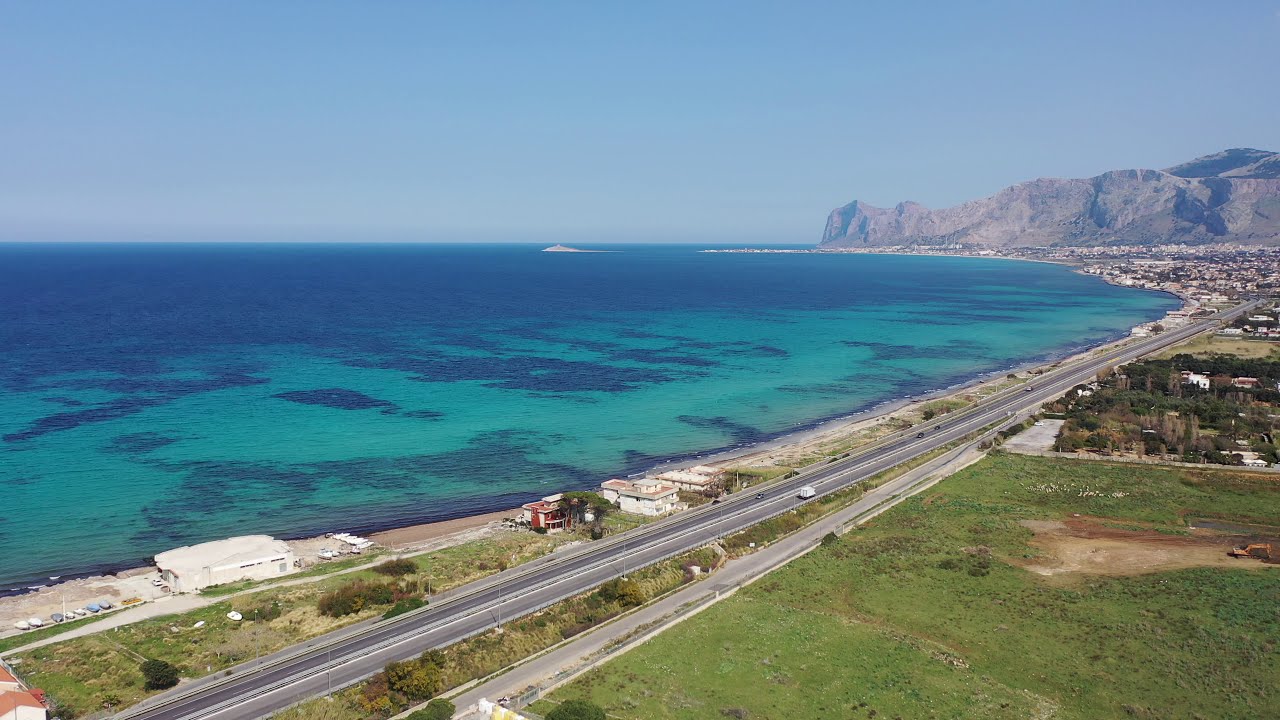The high-angle drone shot captures a stunning landscape where the ocean's crystal-clear, light blue-green water stretches out for miles. Toward the bottom left of the image, a sandy beach fringes the shoreline with parked cars lined up, hinting at public access. A highway bisects the scene diagonally, running from the lower left to the upper right, with sparse traffic. On the beach just beyond the highway, a few older-looking structures, possibly hotels or restaurants from the 40s or 50s, stand with adjacent parking lots. Surrounding these buildings, lush green grass and patches of dirt blend seamlessly into the natural scenery. In the distance, an urban center with widespread development but not many skyscrapers emerges, signifying a transition from the green periphery to a more built-up area. To the upper right, the towering presence of a grayish-brown mountain rises dramatically, creating a cliff-like backdrop that enhances the idyllic coastal setting. The clear blue sky above completes the picturesque view, making this a breathtaking mix of natural beauty and human habitation.